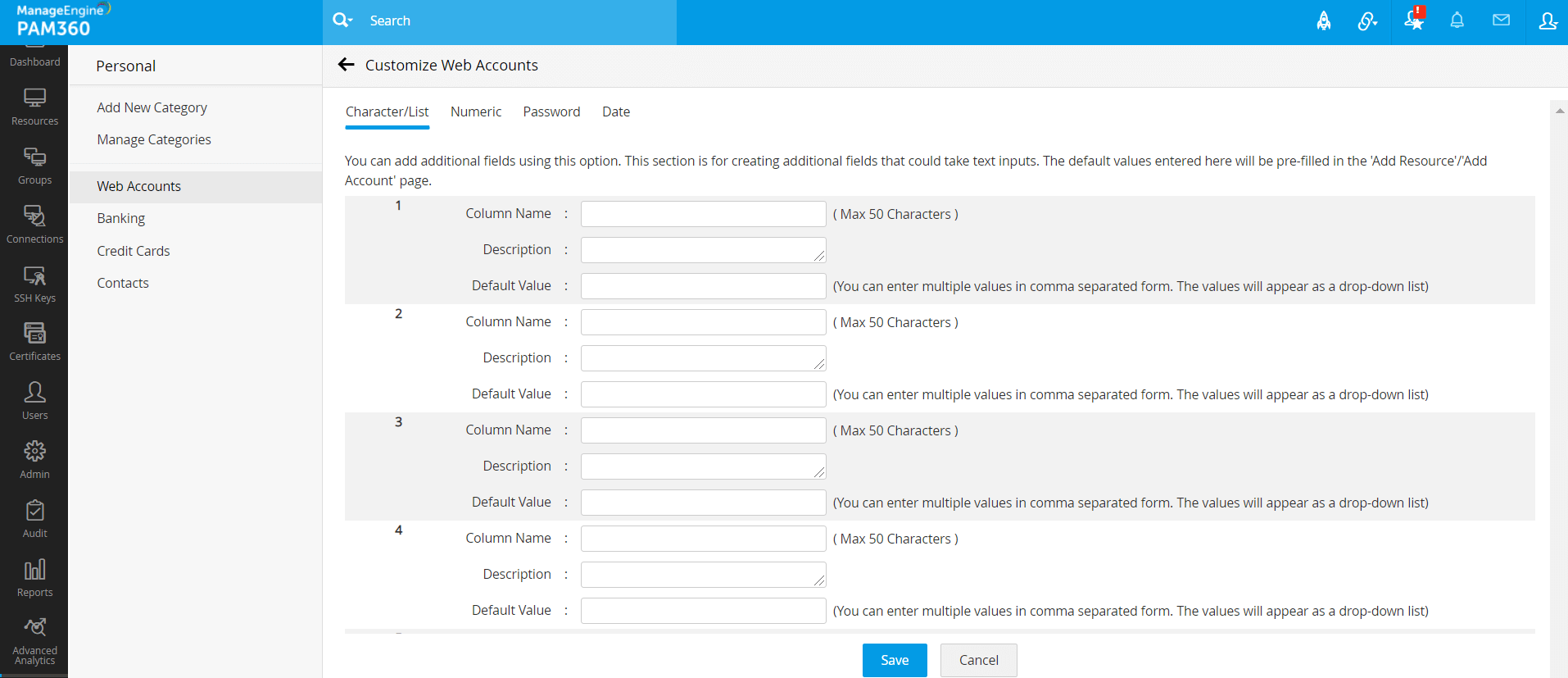The screenshot depicts the user interface of Manage Engine PAM360. On the left side of the screen, a vertical menu displays various tabs with corresponding icons. The tabs listed from top to bottom are: Dashboard, Resources, Groups, Connections, SSH Keys, Certificates, Users, Admin, Audit, Reports, Advanced Analytics. 

Adjacent to this vertical menu is a section titled "Personal." Under this heading, options available include: Add New Category, Manage Categories, Web Accounts, Banking, Credit Cards, and Contacts. The current focus is on the "Web Accounts" tab, which has expanded to reveal the subheading "Customize Web Accounts."

At the top of this customization area are four tabs labeled: Character List, Numeric, Password, and Date. The "Character List" tab is currently selected, indicated by an underlined blue horizontal line. Within this section, users have the ability to add additional fields for text input. Default values entered here will prefill the corresponding fields in the "Add Resource" and "Add Account" pages.

Four subsections are repetitively detailed underneath, each containing fields for Column Name, Description, and Default Value, with a maximum character limit of 50. The interface allows the entry of multiple values in a comma-separated format, and these values will display as a drop-down list for user selection.